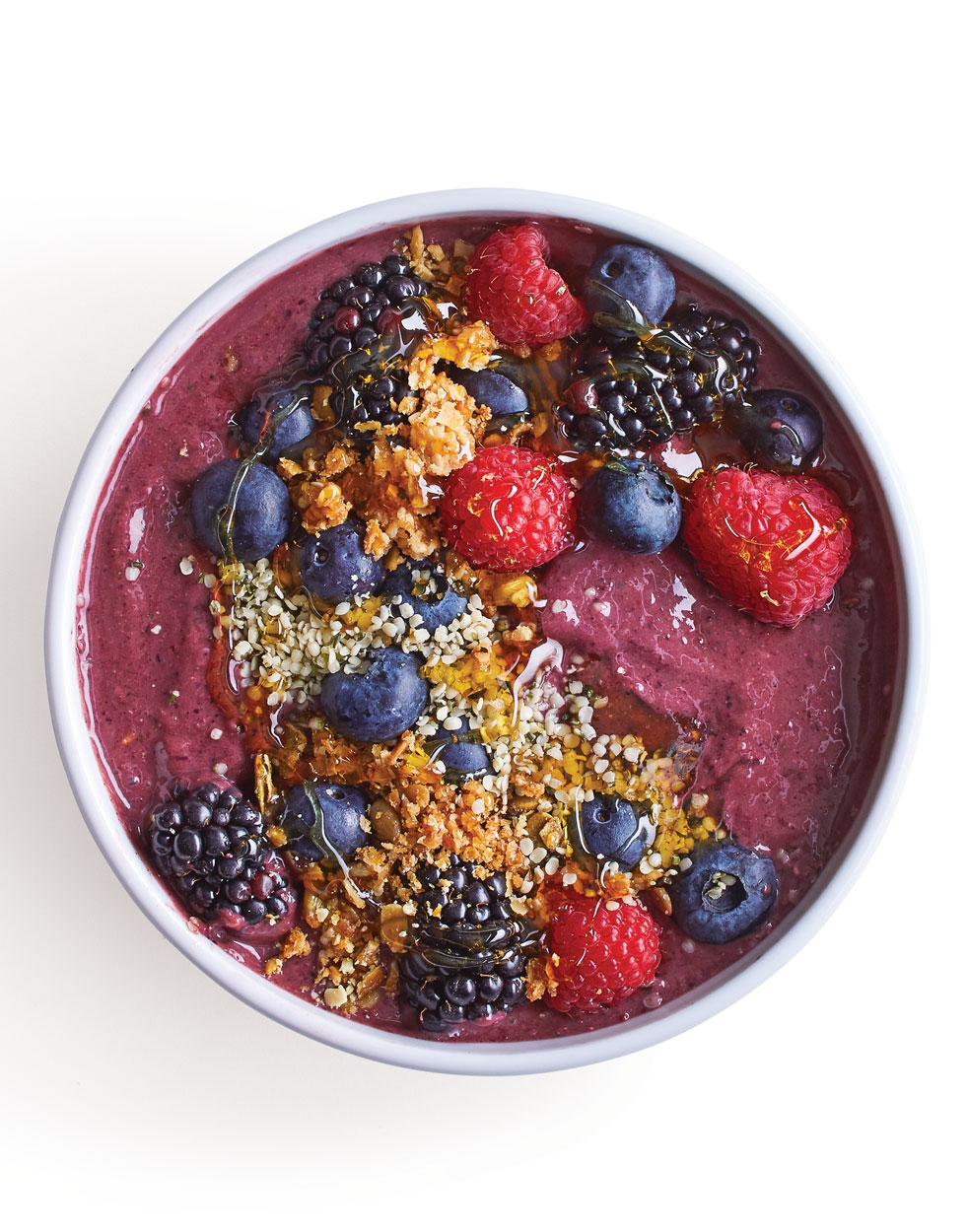This detailed, overhead photograph captures a vibrant and appetizing bowl of acai berry sorbet topped with various fruits and granola. The bowl itself is white with the edge or rim clearly visible against a completely white background, except for a subtle shadow on the left. Inside the bowl, a thick, purple sorbet forms the base, likely a pureed fruit mixture with a firm, pudding-like consistency. This base is adorned with a colorful assortment of fruits, including strawberries, raspberries, blueberries, and blackberries. Sprinkled among the fruits are flaky substances in shades of white and brown, possibly ground granola or seeds such as flax. Additionally, an amber-colored liquid, likely honey, is drizzled over the fruits and granola, adding a glossy and mouth-watering finish to this nutritious and delicious-looking meal, perfect for breakfast or dessert.